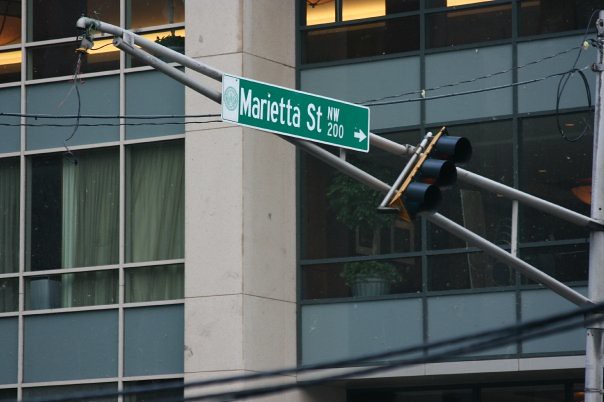The photograph captures a street scene featuring a green street sign that reads "Marietta Street NW 200," with an arrow pointing to the right. This sign is mounted on a gray metal pole, which is part of a triangular support structure. Below the sign, there is a traffic signal, appearing slightly diagonal rather than upright or horizontal. Although the lights of the signal are not visible, black metal covers the areas where the lights would typically be. In the background, there is a commercial building with several windows, one adorned with drapes and another featuring a potted or hanging plant. Electrical cables are strung along the exterior of the building, adding to the urban atmosphere of the scene.